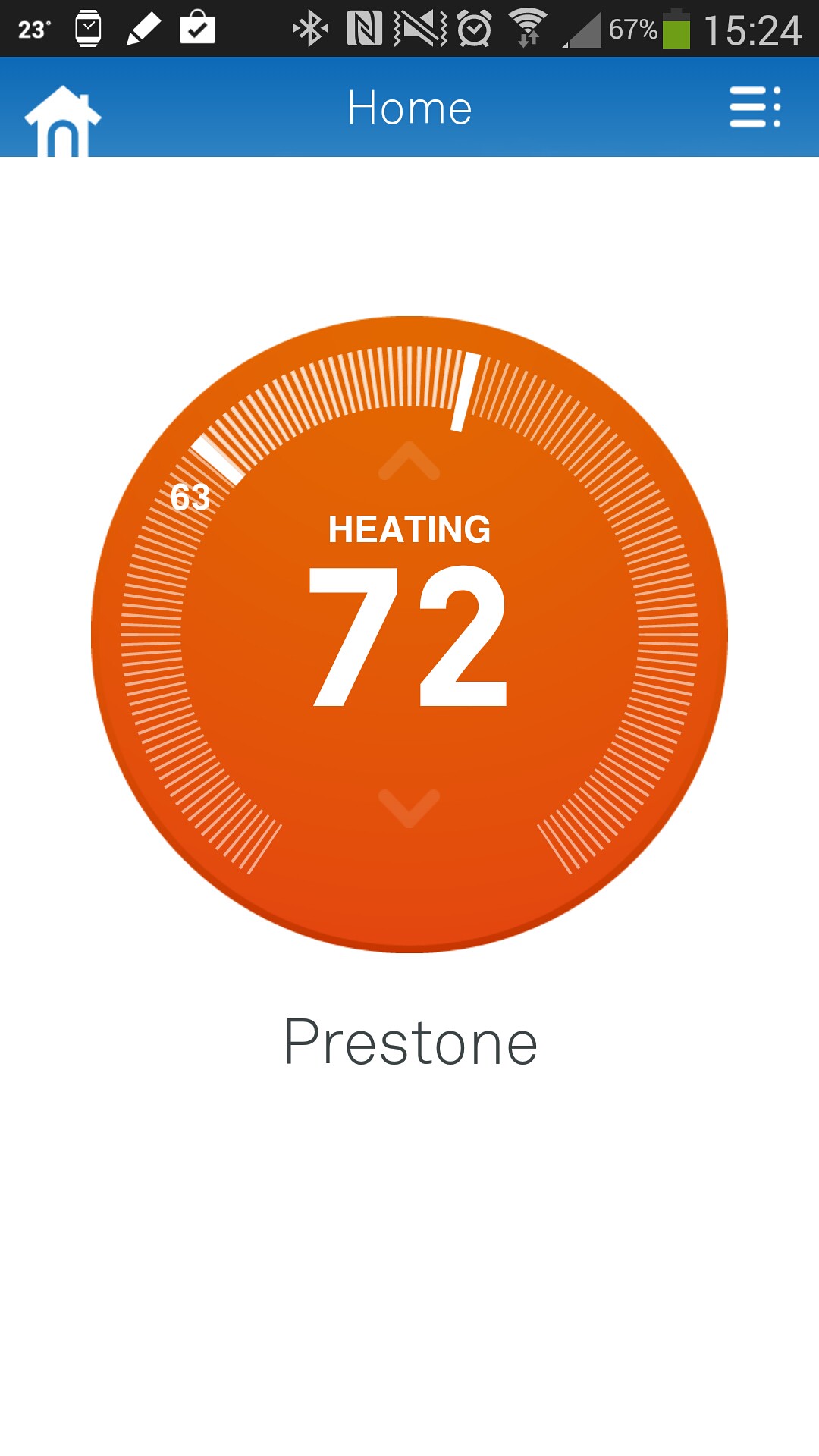This detailed caption describes a screenshot of a cell phone display featuring a home thermostat application:

The screenshot depicts a smartphone screen with an open thermostat app, which is actively managing the home's heating system. At the center of the app's interface, there is a prominent large orange circle displaying the current temperature in white numerals, marked as 72°F. Directly above this number, the word "Heating" is clearly indicated, showing that the heating system is currently operational. Below the orange circle, the label "Prestone" is present. 

At the very top of the screenshot, the phone's status bar is visible, revealing a variety of notifications and status icons: Wi-Fi connectivity, active alarms, Bluetooth status, and the battery level, which is at 67%. The current time displayed is 15:42. Just beneath the status bar, a blue strip prominently displays the word "Home," accompanied by a small house icon to the left, and a drop-down menu icon on the right, indicating additional options available within the app.

Overall, this screenshot captures the interface of the thermostat app, providing clear and detailed information about the home's heating status and other relevant smartphone activity indicators.